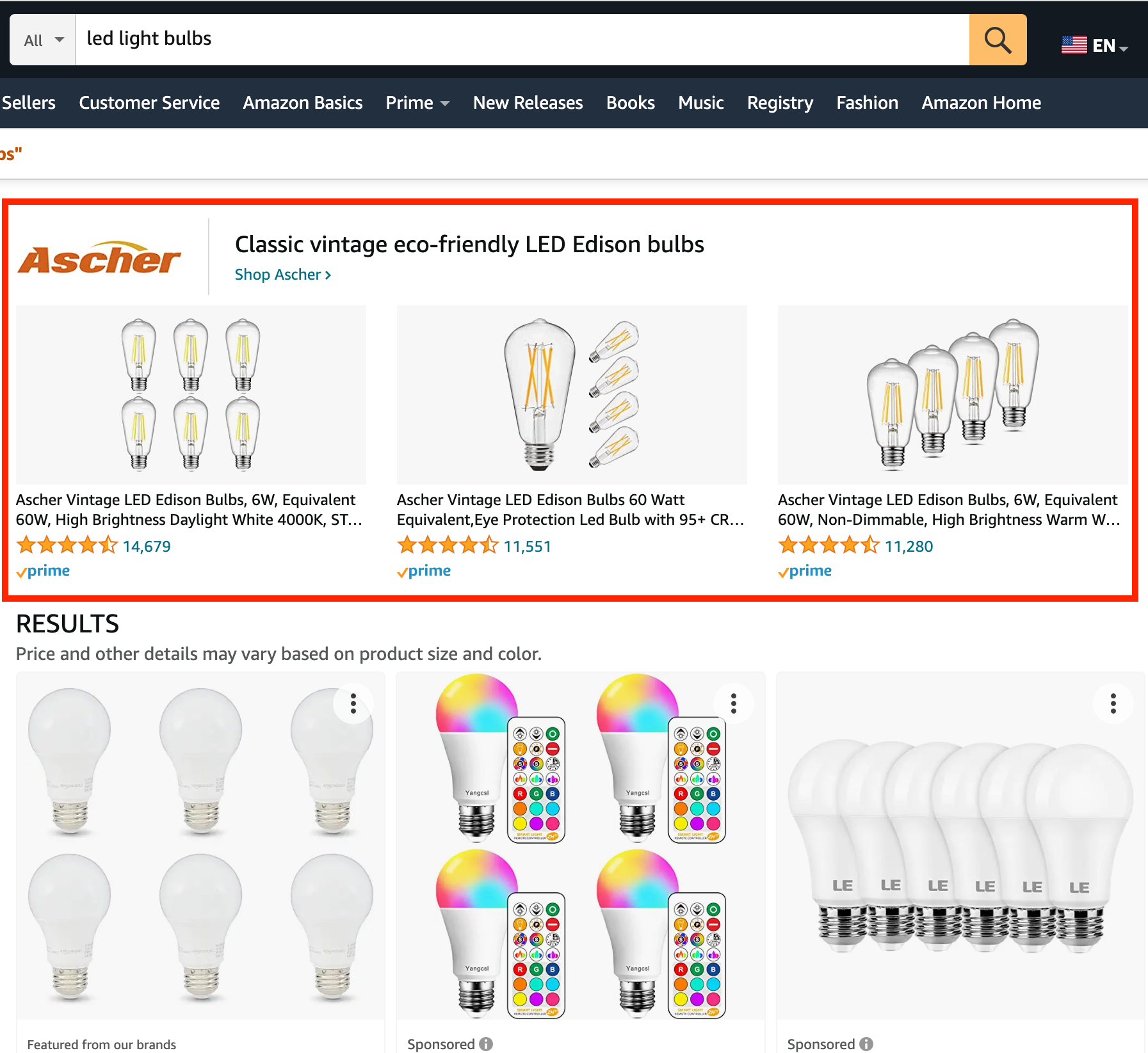This detailed desktop screenshot features a browsing session on Amazon's website, indicating a search for "LED light bulbs." Though the address bar and browser frame are not visible, the Amazon branding and interface are unmistakable. The top right corner confirms the language setting as English. The Amazon menu bar is visible at the top of the screen, displaying links for Sellers, Customer Service, Amazon Basics, Prime, New Releases, Books, Music, Registry, Fashion, and Amazon Home.

A specific product from the company Asher is highlighted in red, displaying their range of Classic Vintage Eco-Friendly LED Edison Bulbs. Three product images are prominently featured:

1. The first image on the left showcases six Asher Vintage LED Edison Bulbs, with a description partially visible that reads, "6 watt equivalent to 60 watt. High brightness, daylight white, 4,000 K." This product has garnered an impressive rating of four and a half stars from 14,679 reviews.
2. The second image displays five bulbs, one of which is larger, possibly for visual emphasis. The description starts with "Asher Vintage LED Edison Bulbs 60 watt equivalent. Eye protection LED bulb with 95 plus CR," before trailing off. This item similarly holds a four and a half star rating from 11,551 reviews.
3. The third image shows four bulbs and begins with "Asher Vintage LED Edison Bulbs 6 watt equivalent to 60 watt. Non dimmable, high brightness, warm," ending abruptly. This product also maintains a four and a half star rating, backed by 11,280 reviews.

Below these images, the screen provides additional browsing options, noting, "Results. Price and other details may vary based on product size and color. Featured from our brands." Further down, it displays a range of bulb types, including traditional white bulbs and a set of color-changing bulbs equipped with a remote control.

The user has clearly initiated a search on Amazon for LED light bulbs, with the focus specifically on various models offered by Asher.